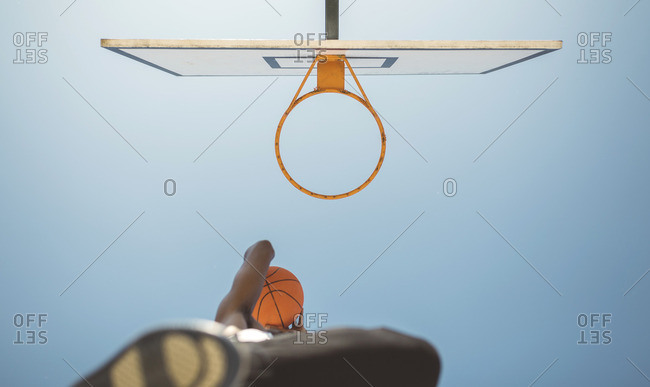This image captures an upward perspective of a basketball player poised to dunk. A prominent, partially blurred sole of the player's shoe occupies the bottom left, with his leg and arm also partially visible, suggesting movement and athleticism. The player, a black man, holds a vibrant orange basketball with black lines, nestled close to his torso. Above him, the hoop appears in a light orange hue, devoid of a net, attached to a white backboard embellished with blue trim. The backboard, supported by a silver pole, features a blue background with a crisscross pattern and inscriptions: "O-F-F" and a reversed "set," centrally marked by the number "0." The overall composition suggests a blend of realistic and possibly computerized elements, emphasizing the dynamic moment before the dunk.